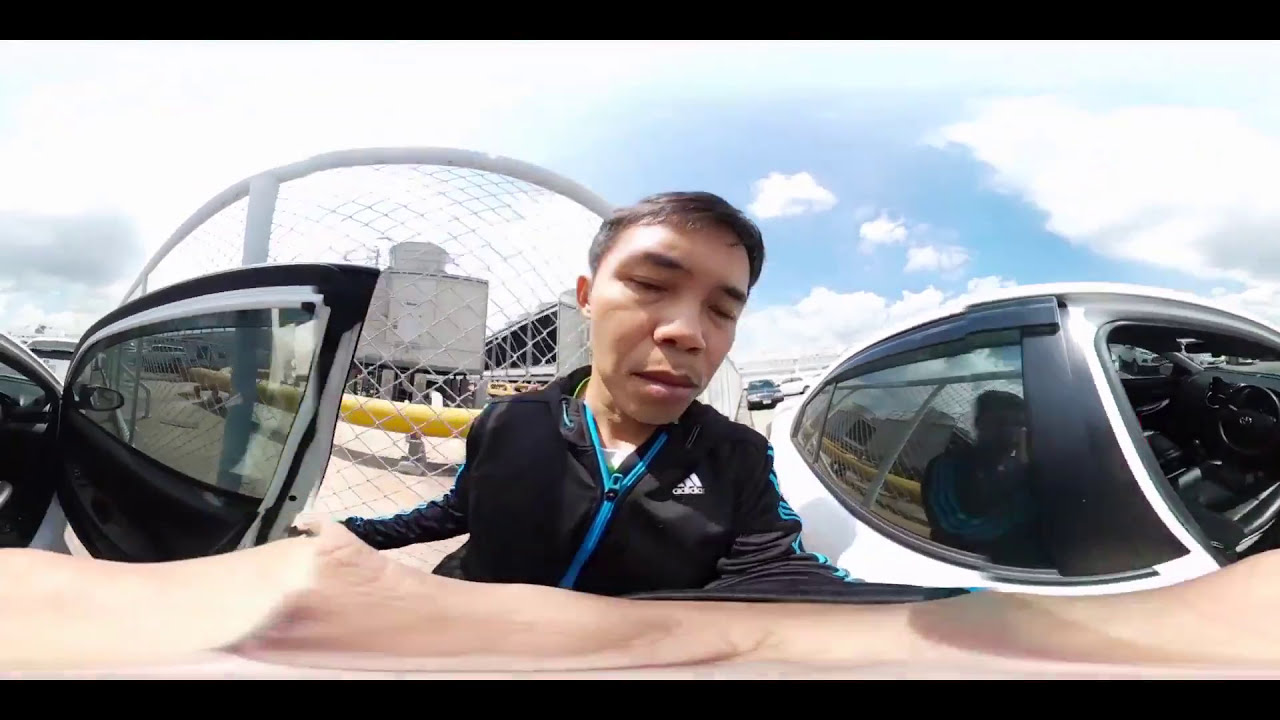The photo captures a wide-angle, fisheye lens shot of a young Asian man in his thirties, standing outdoors on a sunny day with a blue sky dotted by white clouds. He is wearing a black Adidas long-sleeve sweatshirt with the Adidas logo prominently displayed, and a white shirt peeks out from underneath. This man, with short black hair, appears to be in mid-action, possibly entering a car, as his right hand is on a car door. To his left is a car with its door open, facing away, revealing a black interior and some of the white body. To his right is another white car. The fisheye effect distorts the scene, making the cars appear curved and the man's face look larger. The background features a chain-link fence, a yellow railing, gray concrete buildings, and what appear to be industrial air conditioning units, suggesting an industrial or potentially office park setting. The overall ambiance indicates a relatively warm day.